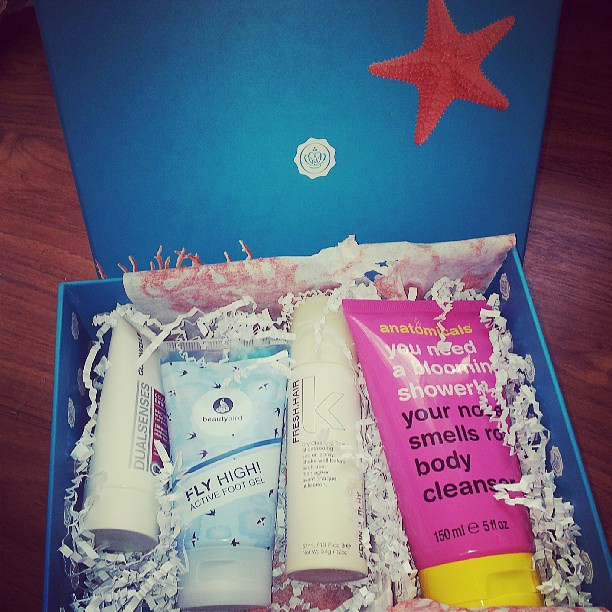The image shows a blue gift box open on a wooden brown surface, likely a table in a house. Inside the box, four personal care items are carefully nestled among shredded white paper confetti used as padding. The items include a pink bottle with a yellow cap labeled "You Need a Bloomin' Shower, Your Nose Smells Something Body Cleanser," a white canister with a partially readable logo featuring a 'K,' a tube of "Fly High Active Foot Gel" adorned with flying bird graphics, and another white tube with the label "Dual Senses." The box is adorned with a white circle in the center, featuring a crown and a wavy edge around it. The blue lid of the box, positioned upright and leaning against something, prominently displays a red starfish in the top right-hand corner and the same central white logo with a crown.